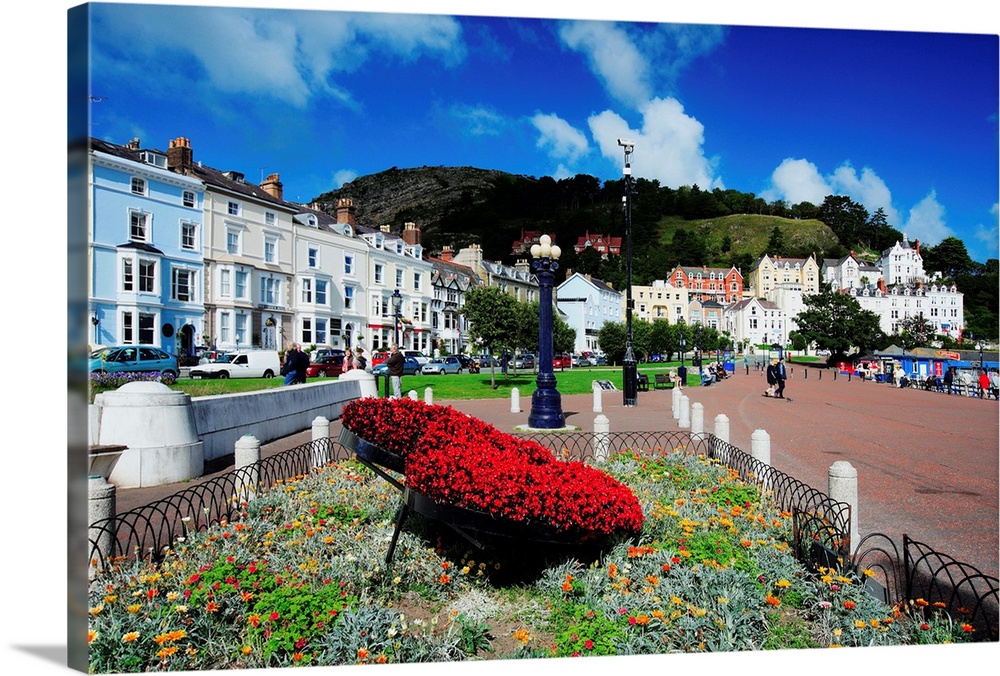This image depicts a vibrant seaside or bayside town beneath a clear, deep blue sky filled with puffy white clouds. A prominent promenade, featuring a long, broad walking path with a reddish-gray hue, runs parallel to the shore. On the pathway, a black metal enclosure houses a large, heart-shaped arrangement of red flowers amid a bed of wildflowers with greens, yellows, and oranges. Beyond this flower bed, two wagons brimming with red flowers add to the vivid scene. The right side of the image reveals a glimpse of water, reflecting the deep blue of the sky.

Surrounding the walkway are patches of green grass and several lampposts. Lining the left side of the promenade are four-story apartment buildings with parked cars in front, suggesting a residential area. These structures, reminiscent of townhouses or condominiums, vary in color from light blue to cream, with a distinct red house perched on a dark hill in the background. Further down the path lies a large white hotel and more apartment buildings. The entire scene is filled with the spirit of a quaint, bustling seaside town, enhanced by the verdant landscape and the picturesque hill topped by buildings.